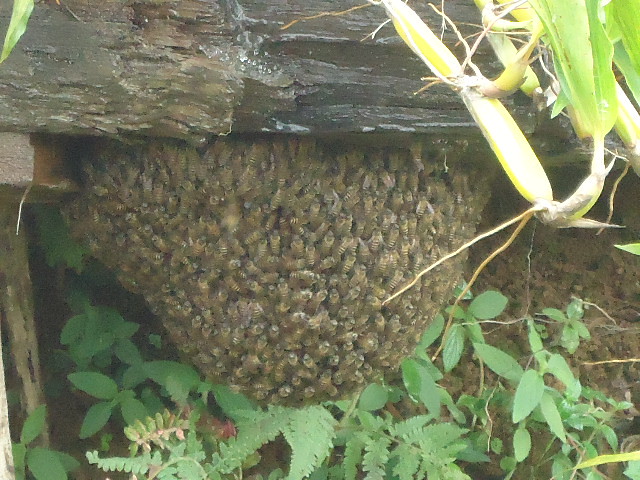This photograph captures a large beehive teeming with hundreds of bees, nestled beneath what appears to be a section of old, dark-colored wood extending from the upper left across to the right before disappearing beneath yellowish-green vegetation hanging down from the top right. The massive hive starts from beneath the wood at the top left, extending downwards and curving to the right, almost reaching the bottom of the image. The bottom part of the hive's arc is rounded, and it tapers off upwards. Surrounding the hive, especially underneath, there is a visible expanse of dirt ground with some leafy green and weed-like plants emerging from the earth. A piece of wood is seen descending beside the hive on its upper left-hand side. The insects populating the hive are numerous, featuring black and yellow striped abdomens and wings, filling the scene with their presence. The meticulous detail in the photograph highlights not only the beehive but also the natural components of its environment, from the aged wood to the modest patches of vegetation and dirt below.